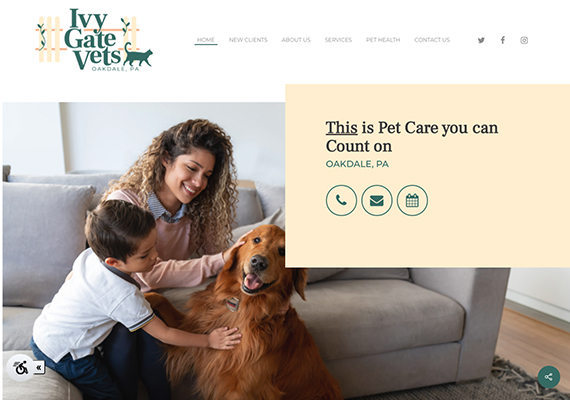This is a description of the homepage for Ivy Gate Vets in Oakdale, Pennsylvania. At the top left corner, the clinic's name, "Ivy Gate Vets," is displayed in dark green text, with "Ivy" on the first line, "Gate" underneath, and "Vets" at the bottom, accompanied by a silhouetted image of a kitten. Behind this green text lies a pink gate design. Spanning across the top, pale gray text includes navigation links labeled "Home," "New Clients," "About Us," "Services," "Pet Health," and "Contact Us." To the right of these links, icons for Twitter (X), Facebook, and Instagram are aligned.

Below the header, a warm, inviting photograph captures a tender moment in a family living room. A mother, with long kinky dark brown hair highlighted, sits on a couch, smiling and displaying dimples. She is dressed in a very light pink crewneck sweater layered over a blue collared blouse. Beside her, her young son, approximately five or six years old, is gently petting an Irish Setter that is cozily nestled on the floor by the couch. The boy places one hand on the dog's chest and another tenderly by its ear. The mother is also petting the dog with a hand placed lovingly on its back.

In the upper right-hand corner of the photo, a light pink box contains the tagline "This Pet Care You Can Count On," underlined for emphasis. Below this tagline, in small, bright blue letters, the location "Oakdale, Pennsylvania" is specified. Adjacent to this text, three icons are displayed within circles: a phone, an email icon, and a calendar, suggesting the various ways to contact or schedule with the veterinary clinic.